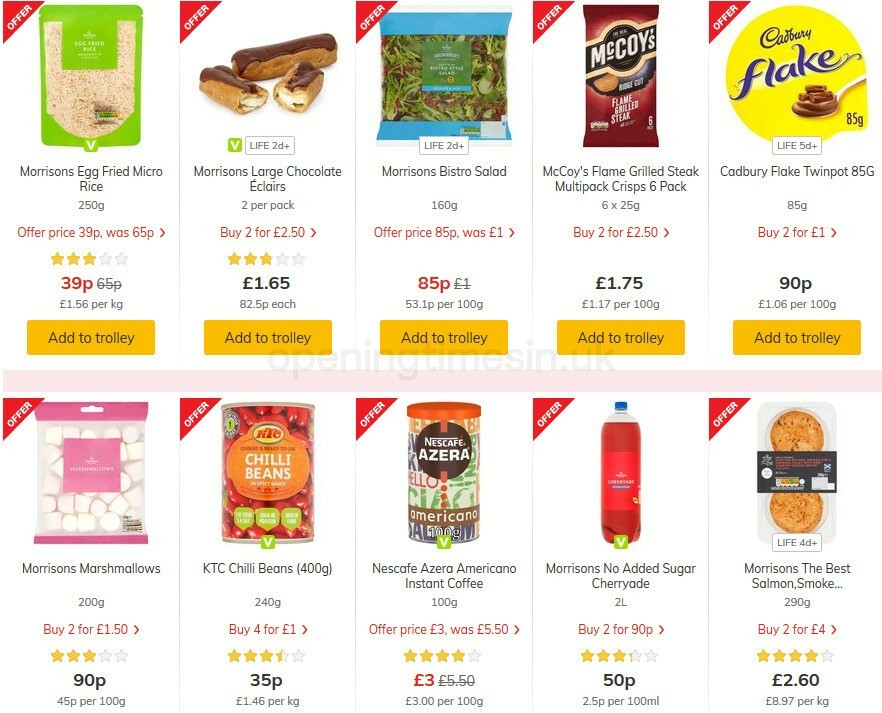The screenshot depicts a webpage from an online grocery store. There are two rows, each containing five columns of product listings. Each product listing features an image of the product, along with a yellow "Add to Trolley" button located at the bottom of the first row's listings, though the text is only visible there.

In the first row, the products featured are as follows (from left to right):
1. Egg Fried Microwave Rice
2. Large Chocolate Eclairs
3. Bistro Salad
4. Flame-Grilled Steak
5. Multi-Pack Crisps

In the second row, the products are:
1. Marshmallows
2. Chili Beans
3. Americano Instant Coffee
4. No Sugar Added Cherry Drink
5. Some kind of Salmon product (details unclear)

The webpage offers a clear and organized layout, facilitating easy browsing and purchasing of groceries.